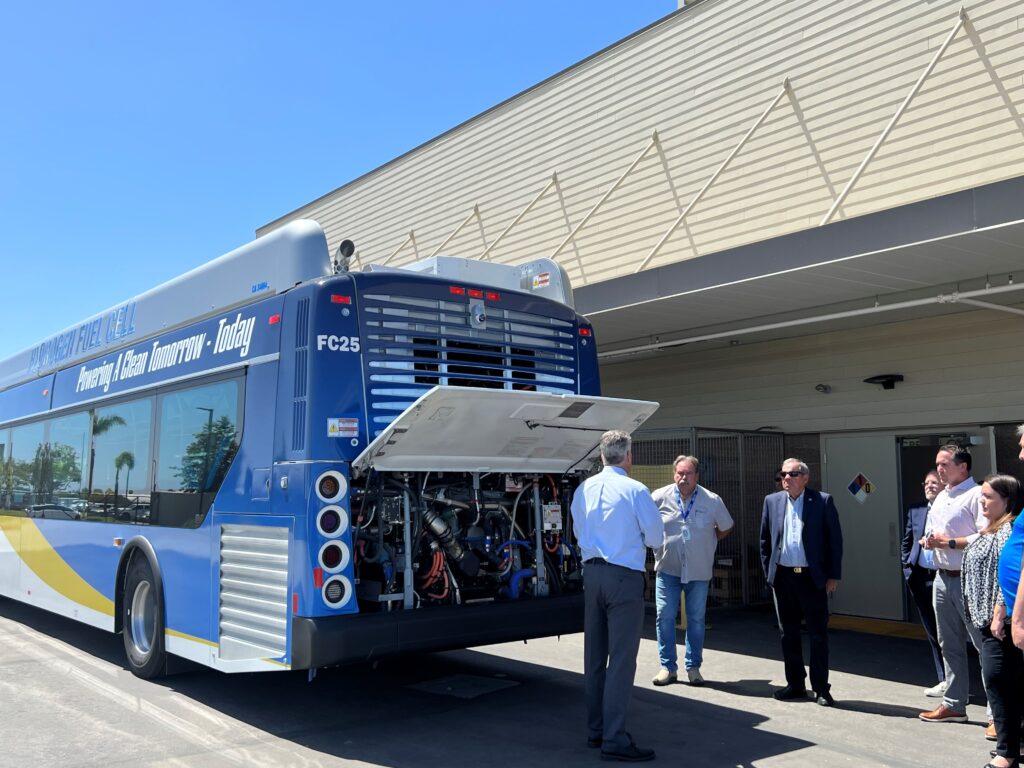This is a detailed color photograph of the rear of a blue city bus with yellow and white stripes, positioned from the middle to the left of the frame. The bus, identified by the number FC25 on the back, has its engine compartment open, exposing various hoses and cables. The rear window showcases louvers and a closed-circuit TV camera, typically used since the driver doesn't have a rearview mirror. The bus displays a white text near the top that reads, "Powering Clean Tomorrow, Today."

A man in a blue shirt and grey pants is standing in front of the opened engine compartment, speaking to a group of seven concerned individuals. The people are gathered on the sidewalk adjacent to the bus, suggesting that they might be passengers facing some mechanical difficulty. In the background, a bus depot with a metallic gray overhang, tan clabbered top, and glass doors can be seen. The overall scene is framed by a clear blue sky visible in the upper left corner, setting the situation in what appears to be a roadside or depot area.